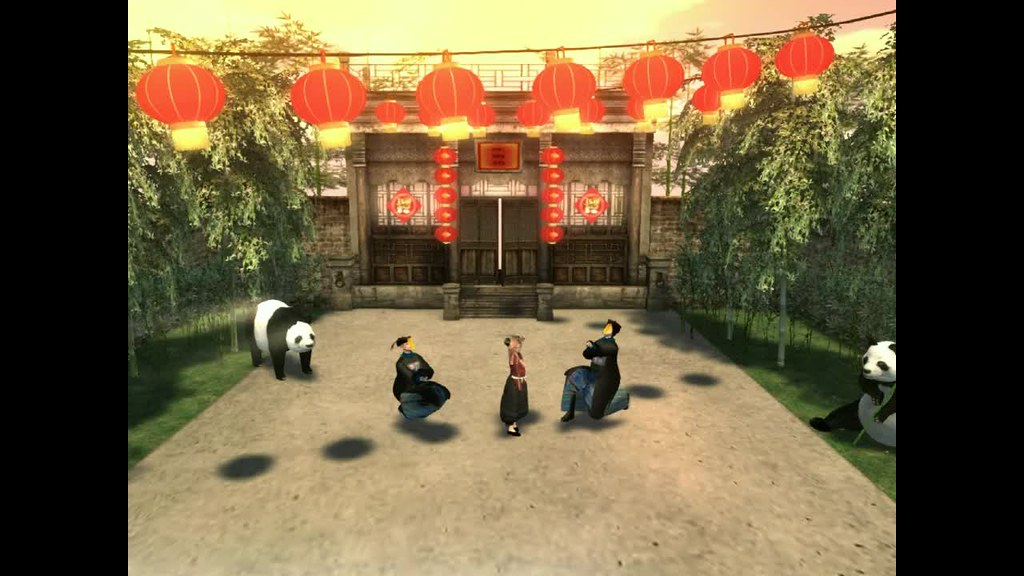This image appears to be a detailed scene from a video game or a piece of 3D rendered digital art with strong Asian influences. The composition is horizontally rectangular with letterbox-style black bars on the sides. At the center of the scene is a serene courtyard, surrounded by brick walls and small grassy areas adorned with trees. In the courtyard are three individuals garbed in traditional, older-style attire—one appears to be a little girl wearing a black bottom robe with a red top, flanked by two adults dressed in long black robes. The characters are either kneeling or squatting.

Dominating the background is a pagoda-like structure with wooden architecture, featuring small stairs leading up to it. This shrine is decorated with numerous large, red, circular lanterns, which hang from a red string stretching across the top of the image. Along the windows of the building are red, diamond-shaped ornaments and two centrally placed doors, all contributing to the traditional aesthetic. 

Additionally, the scene includes two pandas, enhancing the cultural ambiance. One panda is seated on the grass to the right, while the other is walking on all fours from the left towards the group of people in the courtyard. The pandas are framed by eucalyptus trees, adding to the tranquil and authentic atmosphere of this captivating image.